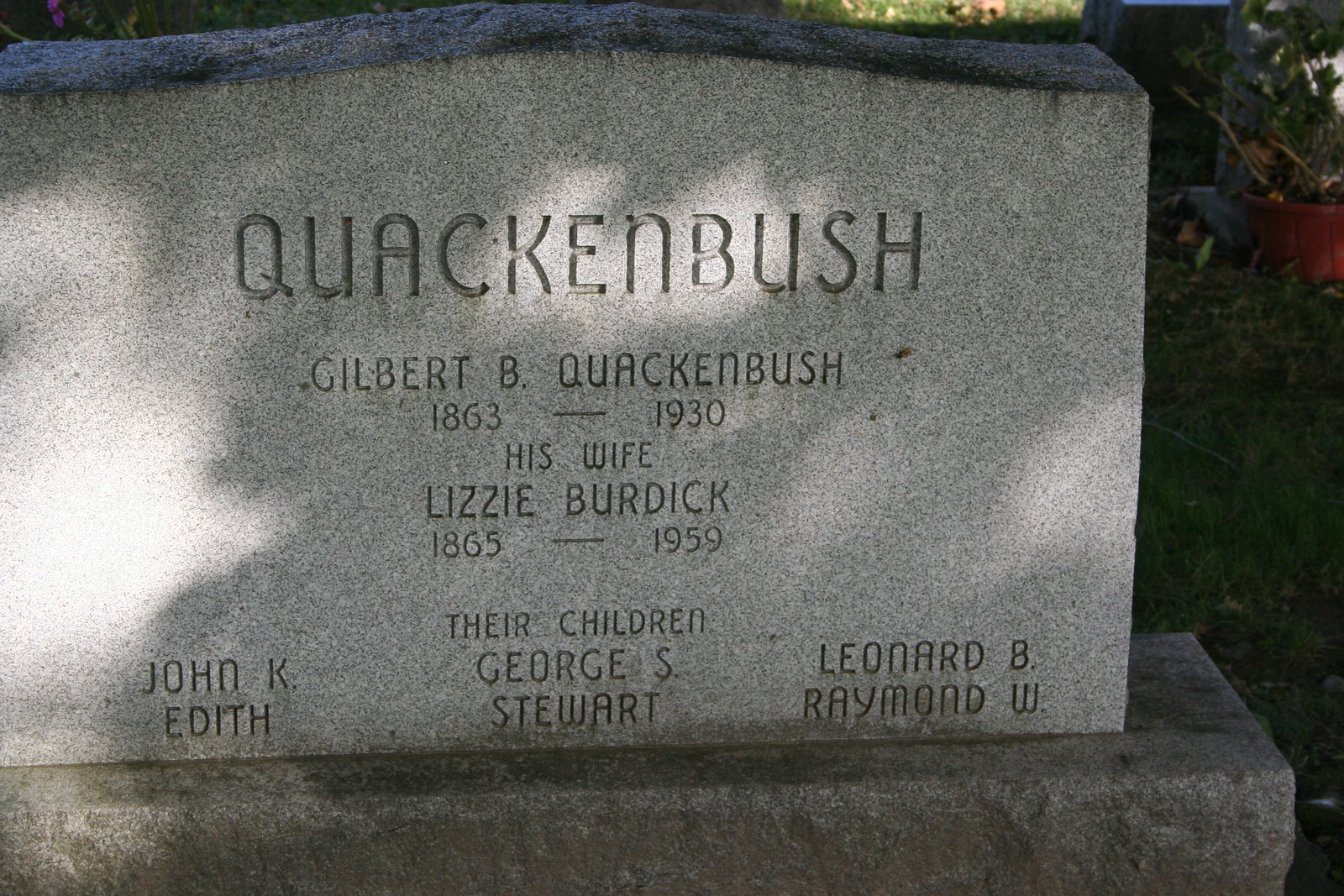This is a detailed outdoor daytime photograph of a gray granite headstone in a cemetery, bearing the surname "Quackenbush" prominently at the top in capital engraved letters. The rectangular tombstone, rounded at the top, is structured on a slightly rougher stone platform. The headstone commemorates Gilbert B. Quackenbush (1863–1930) and his wife, Lizzie Burdick (1865–1959). Below their names, it lists their children: John K., Edith, George S., Stewart, Leonard B., and Raymond W. The background features grass and fallen leaves, typical of a graveyard setting, and to the right of the tombstone, there's a reddish-orange planter with a plant visible.